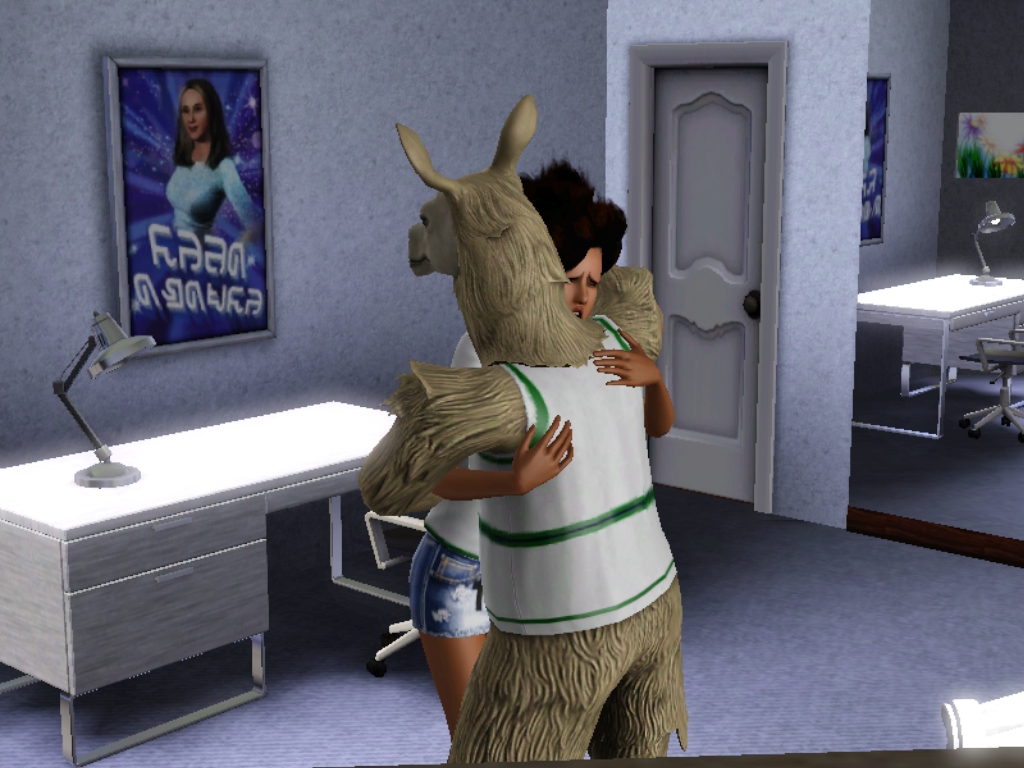This digital, computer-generated image resembles a scene from an animated film or online simulation game. Central to the image is a Caucasian woman with tall, dark hair, appearing distressed, who is wearing a white shirt and short blue-jean shorts. She is embracing a standing llama with light beige fur, which is dressed in a white sleeveless shirt featuring green stripes.

The background reveals a room with gray floors and walls. On the left side, a white study desk with gray wooden drawers houses a silver desk lamp. The desk surface glows brightly, as does a white chair positioned at its front. Above the desk, there is a framed portrait of a brunette woman in a light blue shirt against a space-themed, purplish backdrop. This portrait includes indecipherable foreign writing beneath it.

To the right of the central figures, a gray door is visible near the room's corner. Adjacent to it, a mirror reflects the desk, lamp, chair, and the portrait. This reflection also includes an additional multicolored painting with a white background that doesn’t appear elsewhere in the room. The entire scene is set against a backdrop integrated with elements that blend reality with a digitally animated aesthetic.